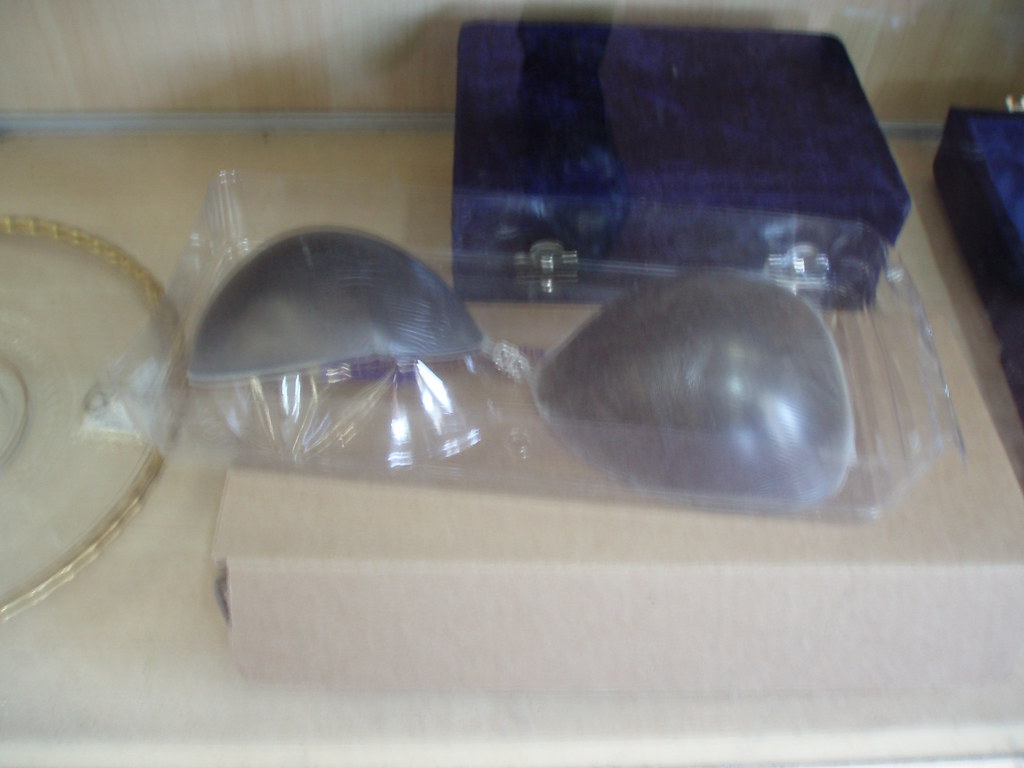In this blurry photograph, a pair of gray, cup-shaped items, resembling the lenses of sunglasses or perhaps a strapless bra, are packaged in a translucent, shrink-wrapped plastic case. These items rest on a shallow cardboard box. In the background, there’s a navy or indigo marbled rectangle, possibly a velvet jewelry box, featuring silver metal clips on both its left and right sides. To the left of the plastic package, there is a porcelain white plate with a gilded edge.